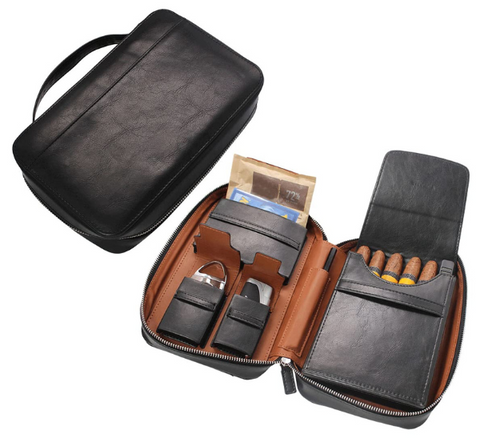This detailed photographic image, set against a white background, showcases a black leather travel cigar case both closed and open. The closed case, displayed in the top left, features a handle and is oriented from the bottom left to the top right. In the bottom right, the open case reveals a well-organized interior with a light to dark brown lining. On the right side, there is a large black pouch containing five yellowish cigars with brown tips. To the left, the case includes three smaller pouches: the top pouch appears to contain papers, the middle pouch likely holds a cigar cutter, and the bottom pouch contains a silver and black cylinder whose purpose is unclear. This thoughtfully arranged layout highlights the case's functionality for securely storing and transporting cigars and associated accessories.